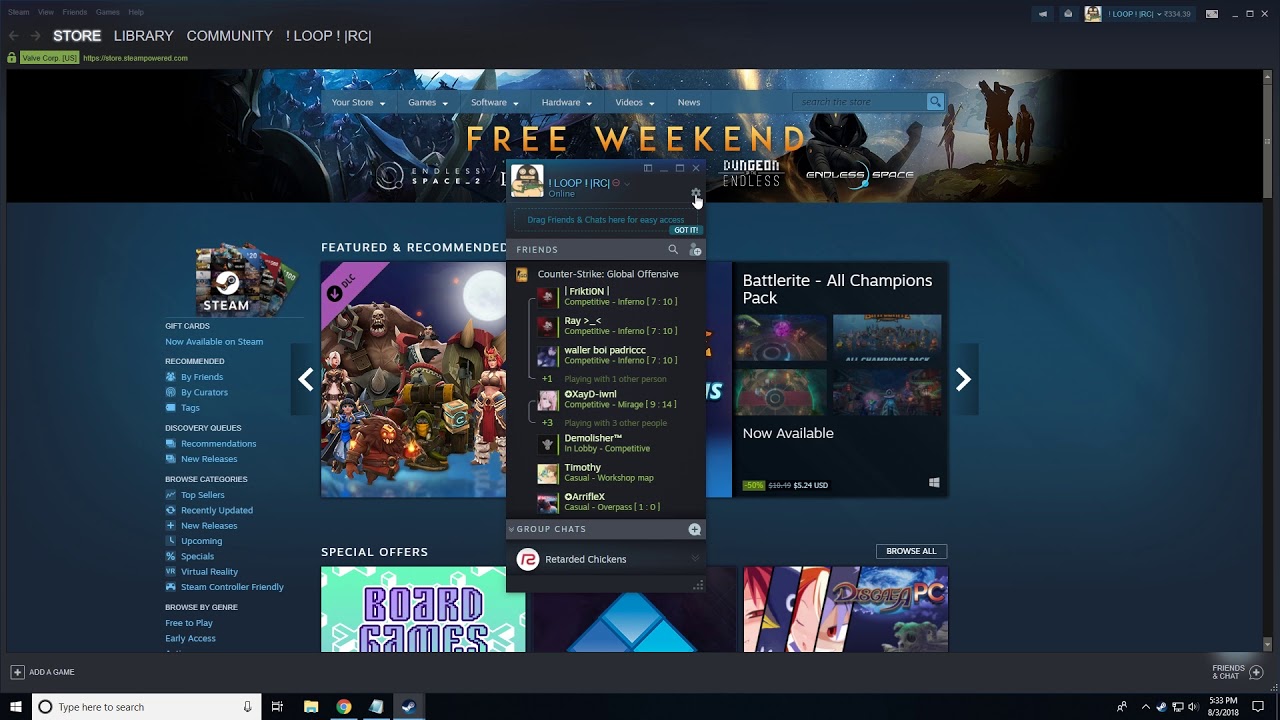Screenshot of the Steam Launcher for PC

This screenshot captures the main interface of the Steam Launcher for PC. In the top left corner, we can see the prominent menus labeled 'Store,' 'Library,' and 'Community.' These are followed by a secondary menu, 'Loop RC,' though its specific function isn't immediately clear. 

Dominating the upper portion of the launcher is a horizontal banner with the words "Free Weekend" prominently displayed. Positioned above this banner is another smaller menu, featuring options such as 'Videos' and 'News', although they are somewhat difficult to make out clearly.

On the left side of the main portion of the launcher, there is an image representing Steam Gift Cards. Directly beneath this image lies a vertical menu with options like 'Recommend', 'Option', and 'Browse Categories'.

At the center of the launcher, several game titles are featured and recommended for the user. Notably, the "Battlerite All-Champions Pack" is prominently displayed among these recommendations.